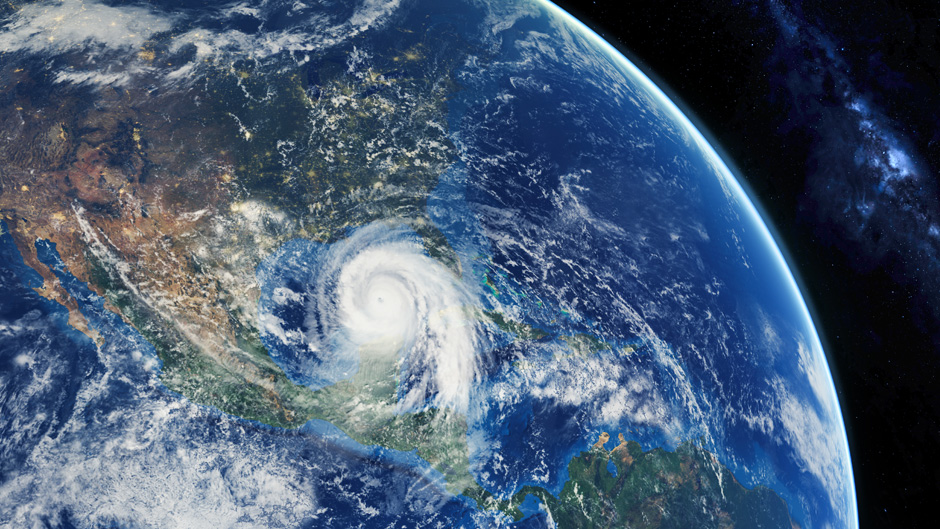The image displays an overhead view of Earth from a satellite, focusing on the Gulf area of the United States. Dominating the Gulf is a massive, white spiral hurricane that pretty much occupies the entire region. The image captures extensive geographical details including Central America, most of the United States, the northern part of South America down to Brazil, and both the Atlantic and Pacific Oceans. The bodies of water appear dark blue, while the continents showcase a dark green and brown palette, indicating varied terrain and mountainous areas. To the right of the image, the blackness of outer space is punctuated by a visible galaxy or star cluster, adding depth to the celestial backdrop. The curvature of the Earth is adorned with a faint white glare, enhancing the image's realism and the celestial theme.